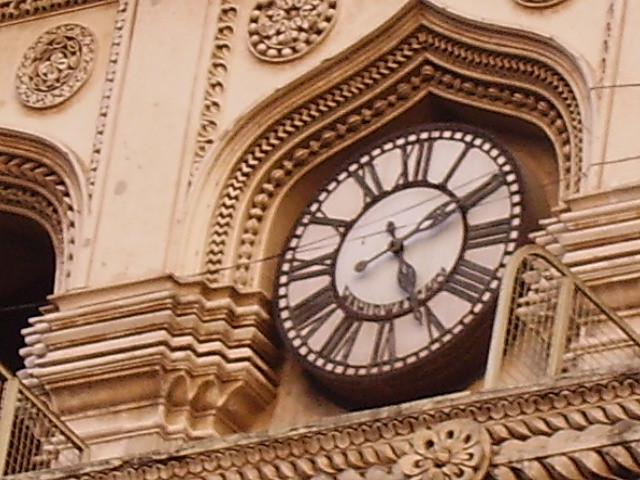The image showcases the upper portion of a tall, ornately designed building, featuring an intricately detailed clock set into an alcove. The clock, displaying the time as 5:10, is crafted with Roman numerals in dark brown against a tan background. Surrounding the clock are elaborate architectural elements, including patterns that gracefully curve and fine embroidery-like details, suggesting the building may have some governmental or institutional significance. The perspective of the image captures the viewer's gaze upward, focusing on the exquisite craftsmanship of this small, yet prominent section of the building.